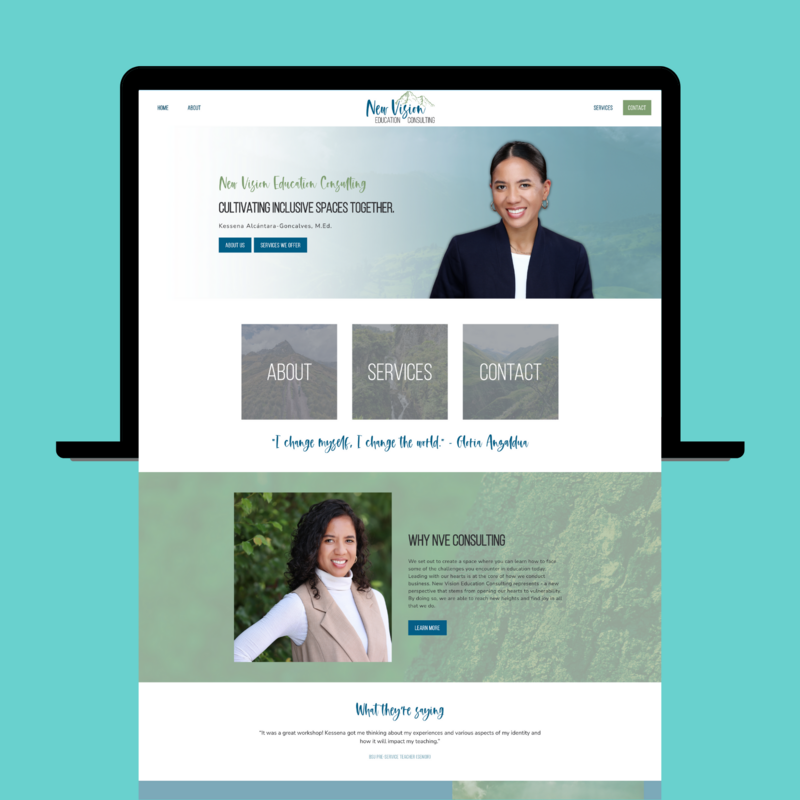This screenshot from a website features a mint green card with two distinct sections. The top section is bordered by a black line that outlines a path from the center left, moving right, up, over, down, and then right again, mimicking the appearance of a web page.

At the top of the webpage, the navigation menu includes options such as "Home," "About," "New Vision," and an unreadable option in the upper right corner. Below this navigation bar is a large banner image with a marbled background in light blue and green hues. The image prominently displays a woman with tan skin and black hair pulled back, wearing earrings, a white shirt, and a black jacket. 

On the left side of this image is text that starts with "New Virgin Education..." followed by phrases like "cultivating inclusive spaces together." Two blue buttons are visible beneath this text.

Below the main banner, still within the black-bordered area but set against a white background, are three blocks labeled "About," "Services," and "Contact," each featuring blurred nature scenes in the background. Beneath these blocks, in blue text, is an inspirational quote: "I change myself, I change the world" attributed to Gloria Angaldo.

The bottom section of the card features a darker green area showcasing a darker-skinned woman with black hair alongside the text "YNVE Consulting" and a heading, "What They're Saying."